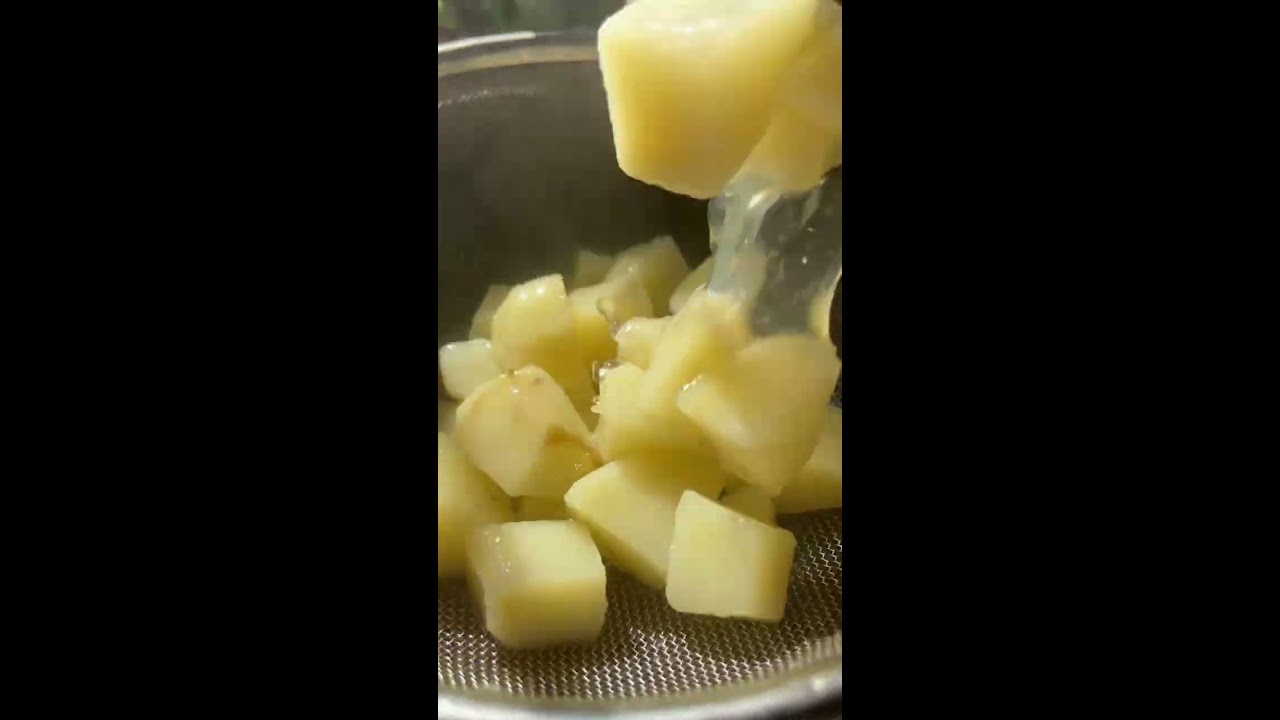The image is a vertical photograph featuring a small silver-colored metal strainer filled with moist, reflective chunks of light yellow fruit, resembling pineapple. There are large vertical black bars on both the left and right sides, which occupy majority of the image, highlighting the central scene. Inside the strainer, the fruit pieces appear in square and triangular shapes, with a particularly large chunk hovering just above the top right section, about to fall in. This piece has a slimy yellow liquid cascading down its side, forming a thick stream that takes up about 25% of the photo's width. The light reflecting off the moist fruit indicates a wet surface, emphasized by the steam rising, suggesting the water is scalding hot. The entire setup is brightly lit from above, capturing the glossy texture of the fruit and the reflective surface of the strainer.